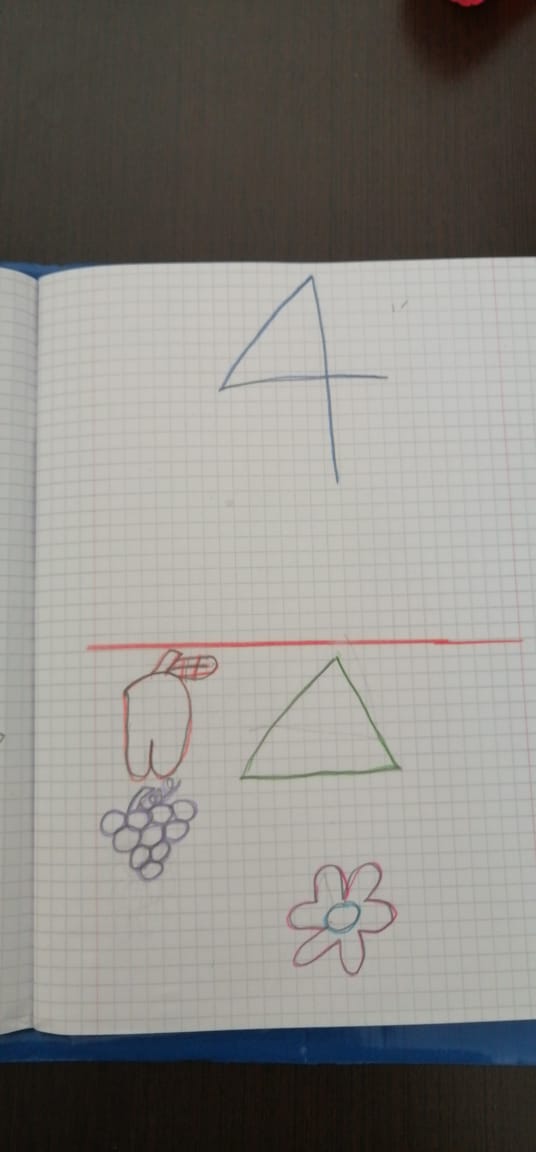The image features a close-up of a grid notebook page placed on a dark, round wooden table, partially backed by a dark blue piece of construction paper. The lighting in the room is low, casting shadows and giving the white grid paper a dim appearance. At the top of the page, a prominent blue number "4" stands out. About halfway down, a horizontal red line spans the width of the paper. Below this line, several colorful shapes and sketches are visible. 

First, there is a red apple complete with a red leaf featuring a small hash mark. Adjacent to the apple is a green triangle. Further down the page, a cluster of purple grapes, detailed with a stem and leaf, can be seen. To the right of the grapes, there's a drawing resembling a flower, with a blue circular center and red petal-like shapes that curve up and down, reminiscent of noodles. The detailed arrangement of these shapes and colors suggests a theme of various figures or objects, unified by the red dividing line.